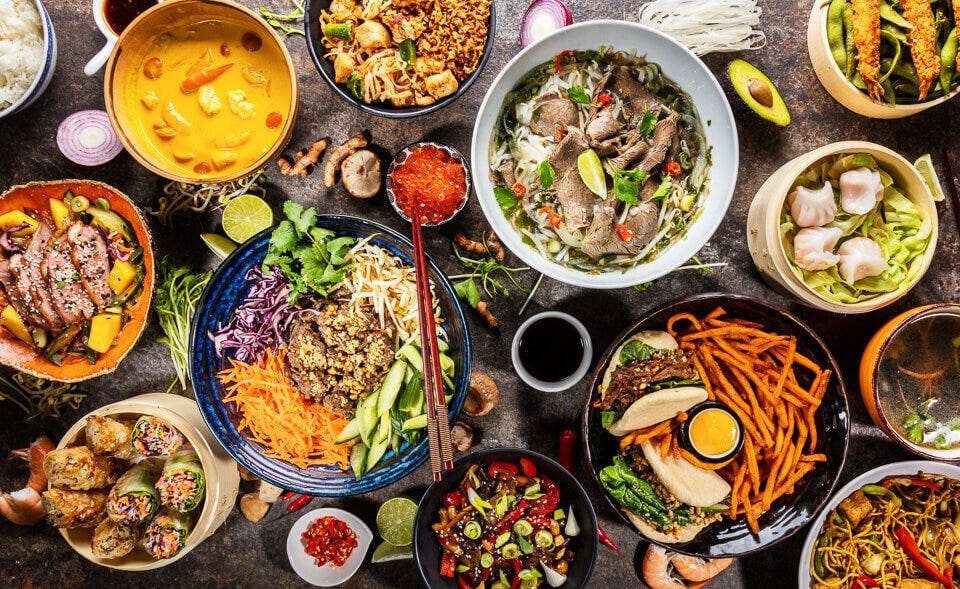The image showcases an impressive and vibrant spread of various Asian-inspired dishes set against a dark gray surface. The table is completely covered with a plethora of foods, presented in an assortment of colorful dishes—blue, white, black, orange, and more. Central to the spread are distinct elements like banh mi sandwiches filled with meat and accompanied by french fries, fried noodle dishes like lo mein, and vibrant green bok choy. Various steaming baskets reveal dumplings, spring rolls, and cabbage rolls, adding to the feast.

A close inspection reveals a range of additional items like cut avocados, halved onions, and an array of citrus fruits interspersed across the table. The presence of several root vegetables, such as sweet potatoes and regular potatoes, accompanied by meat dishes coated in sesame seeds, adds to the diverse texture and flavor profile of the spread. Sauces in hues of yellow and rich tomato-like red are spotted throughout, along with cups of relishes and bright ginger.

Some dishes stand out for their intricate presentation and unique ingredients: a bed of bok choy cradling pot stickers, a tantalizing orange soup, and a refreshing bowl containing cabbage, carrots, cucumber, bean sprouts, cilantro, and an intriguing unidentified ingredient. Adding to the variety are ramen dishes with meat, a tuna mango creation, and the unmistakable presence of chopsticks hinting at the Asian authenticity. The eclectic array of vegetables, from broccoli to carrots to cucumber, complements the proteins—shrimp and prawns, providing a bounty of colors and flavors. This spread is a celebration of vibrant, diverse, and richly textured Asian cuisine.